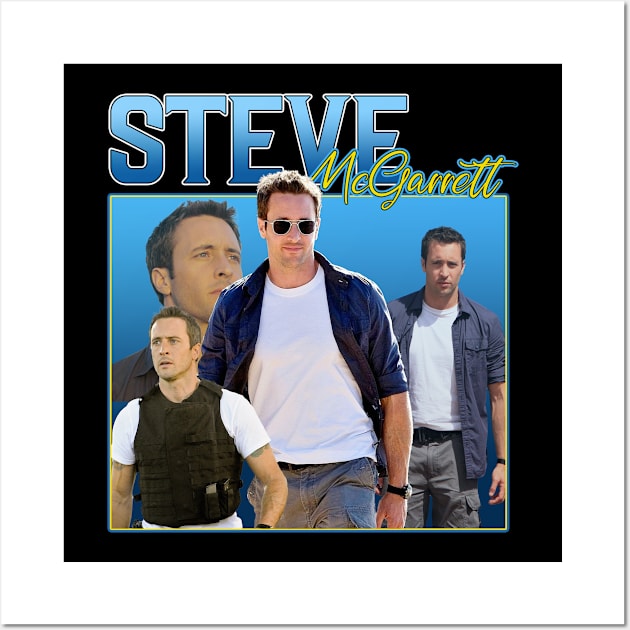The image displays a square poster with a thick white border and a black background. At the top, the name "Steve" is prominently written in large blue capital letters, while "McGarrett" appears in a smaller, yellow cursive script. The central focus is a vibrant yellow square with a blue background, showcasing a collage of four overlapping photographs of Steve McGarrett, a white man with light dark hair and sideburns, who may be an actor or a character. In the central image, he is wearing a white t-shirt, a black jacket with rolled-up sleeves, and sunglasses. The bottom left photograph features him in a white t-shirt and a bulletproof vest, looking intense. The photo on the left shows him glancing upwards, perhaps at the sun, while the one on the right captures him standing and looking directly at the viewer, dressed in a white shirt with rolled-up sleeves.